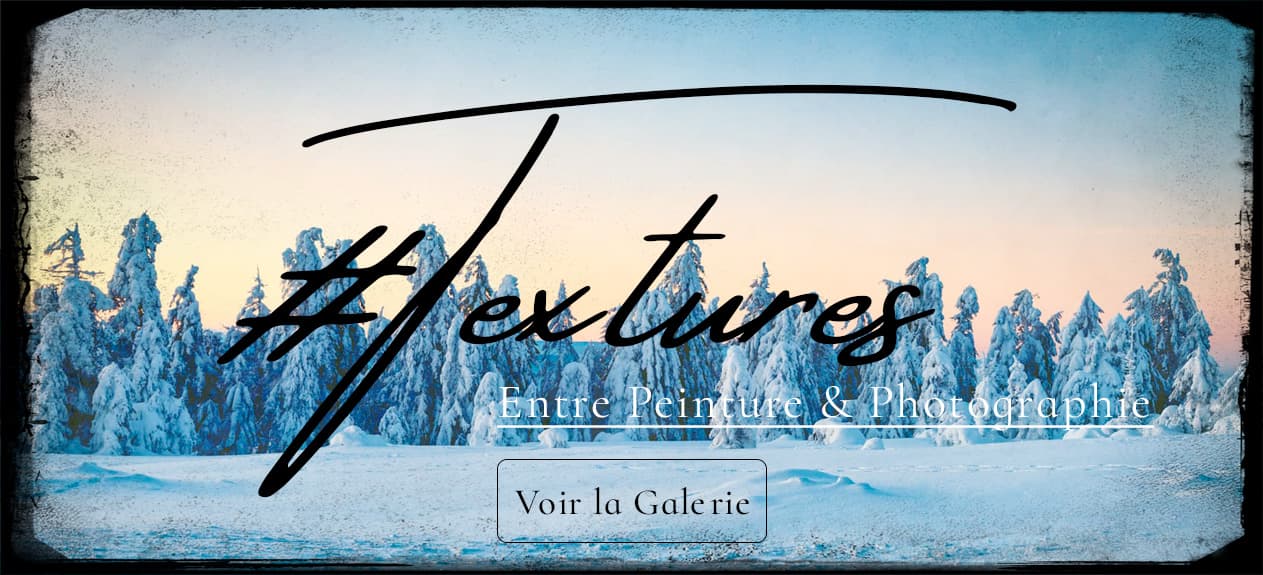A full-color, rectangular horizontal photograph captures an enchanting winter scene outdoors, likely around sunrise or sunset, evidenced by the gradient sky transitioning from a yellowish glow at the horizon to a deep blue above. The natural landscape prominently features a forest of snow-covered pine trees of varying sizes, standing in front of rolling snowdrifts that hint at the considerable snow depth. The entire image is framed by a thin, slightly smudged black border, adding a touch of artistic presentation. 

Centrally placed across the photograph in large, cursive writing is the hashtag "#textures," emphasizing the varied tactile elements of the scene. Below this, in a traditional print font in white, are the words "Entree, Pinture, and Photography," giving the impression that this is an advertisement for an art gallery. Further down, in small black rectangles, the French phrase "Voir la Galerie" invites viewers to explore the gallery's offerings. The combined textual elements and the serene, snowy landscape create a captivating visual narrative that merges natural beauty with artistic expression.